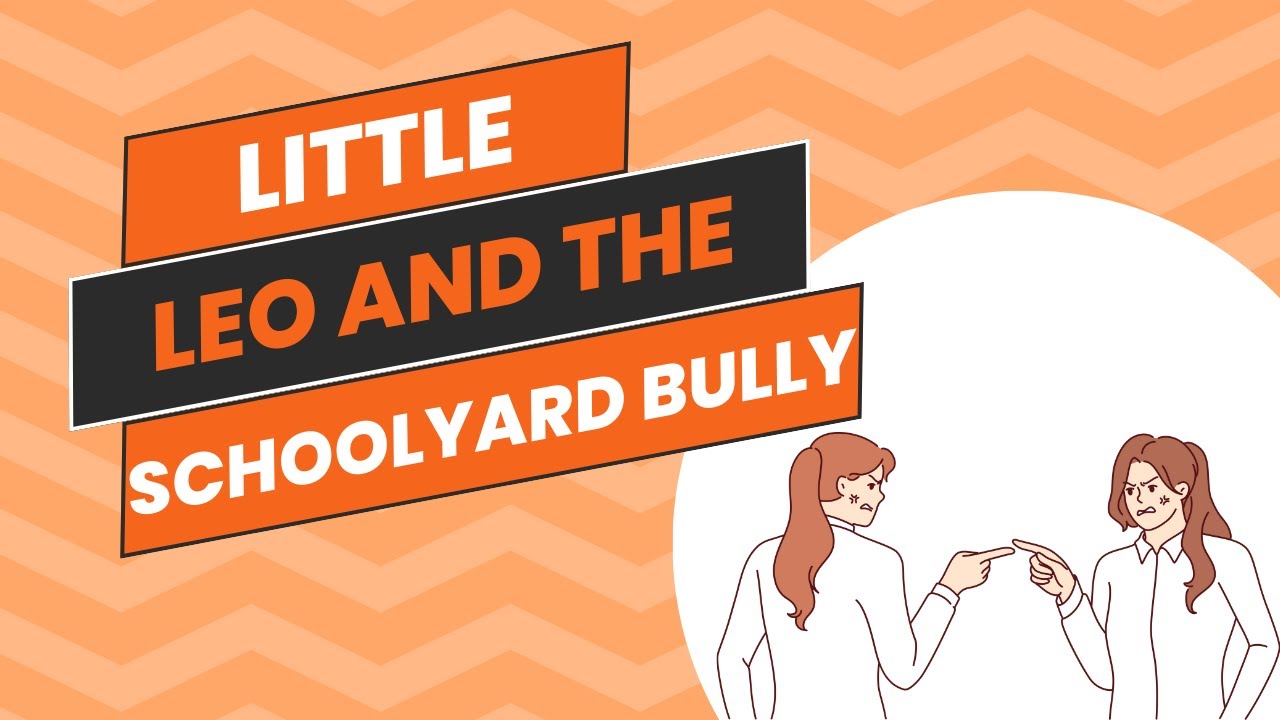This illustrated image appears to be a flyer, likely promoting a book titled "Little Leo and the Schoolyard Bully." The title text is creatively placed on the left side of the image, with "Little" and "Schoolyard Bully" rendered in white font within orange rectangles that have black borders, and "Leo" and "the" displayed in orange font within black rectangles that have white borders. The background is a chevron pattern consisting of alternating light and dark orange stripes.

In the bottom right corner of the image, there is a prominent white circle enclosing an illustration of two women who appear to be in the midst of a heated argument. They are both dressed in white shirts and have light brown or reddish-brown hair pulled back into ponytails. The women are angrily pointing fingers at each other and each has a visible bruise on her face. This visual element likely underscores the conflict theme central to the book's message about dealing with bully behavior in school settings.